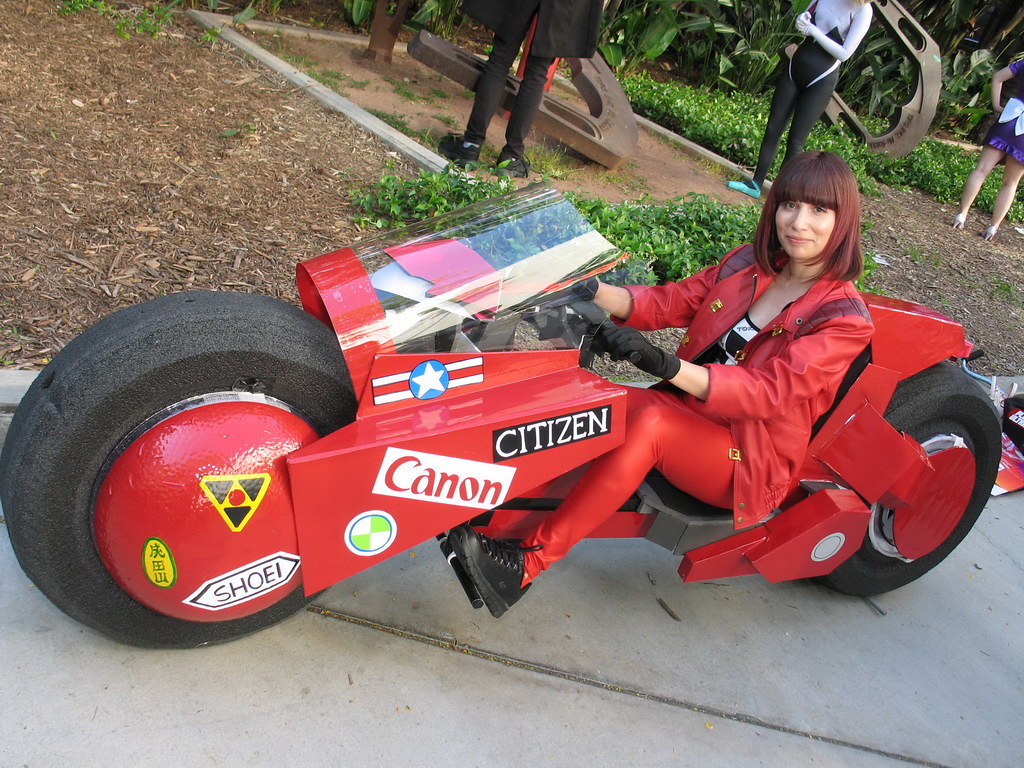In this vibrant image, a woman with red-tinted bobbed hair is captured riding a strikingly low-to-the-ground, futuristic motorcycle, which seemingly resembles a fusion between a motorcycle and a go-kart. The entire vehicle is a vivid red, adorned with numerous logos and decals including "CANON" in red letters on a white background, "CITIZEN" in white letters on a black background, and "SHOEI" in black letters on a white label. Additionally, the motorcycle showcases a variety of intricate symbols: a white circle with green triangles, a yellow triangle housing three black triangles with a red circle in the center, and an oval featuring Chinese characters. Notably, a patriotic touch is added with an American flag symbol, consisting of red and white stripes with a blue circle and a white star.

The woman, possibly of Indian or Latino descent, is dressed in matching red attire—a red jacket over a black and white top, red pants, black gloves, and black shoes—complementing the motorcycle's aesthetic. She is smiling directly at the camera, exuding a sense of excitement and pride. Behind her, a park setting unfolds, with a grassy area populated by people who appear to be in costumes and scattered art exhibits, including iron statues, enhancing the scene's lively and artistic atmosphere.